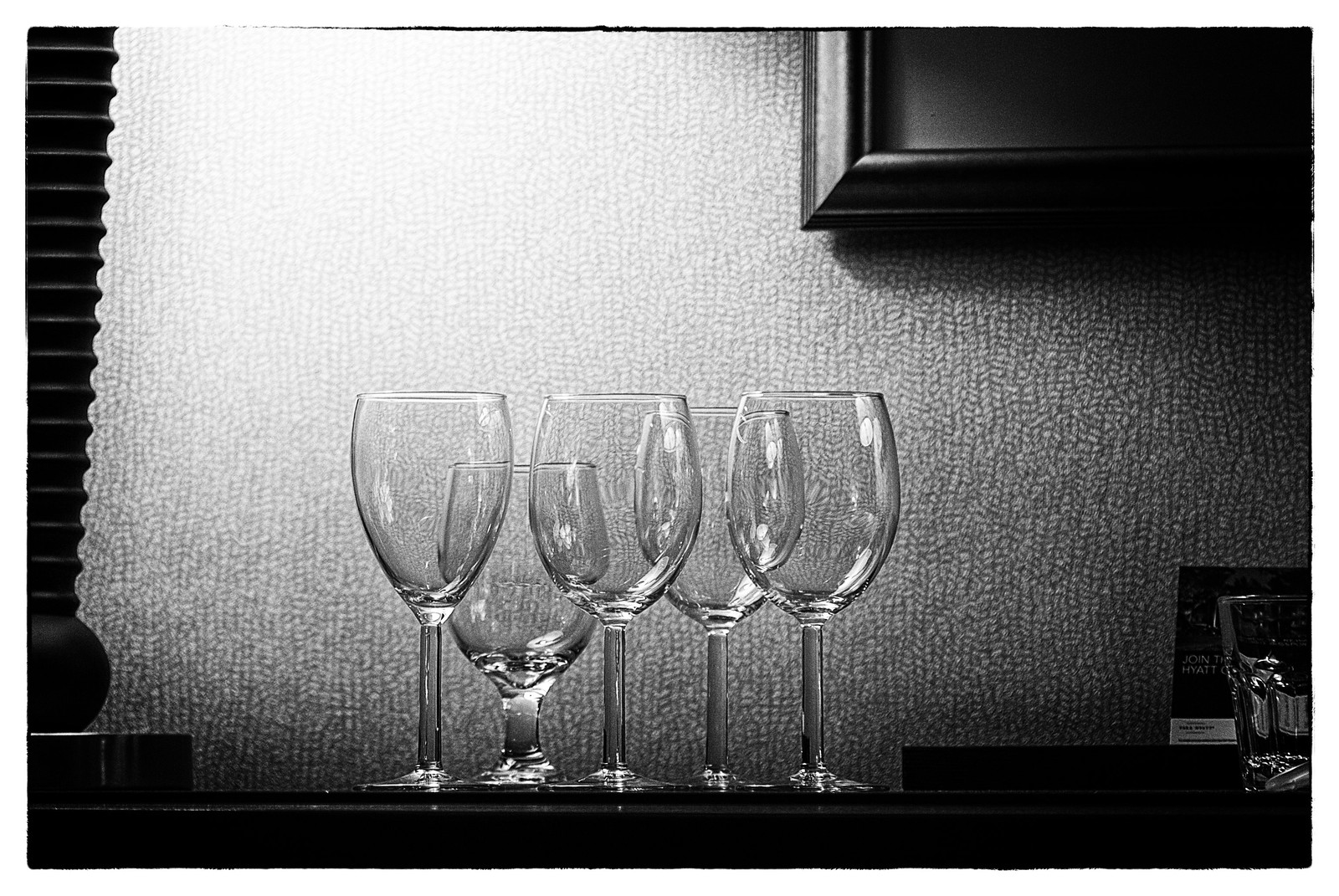The black and white photograph captures a striking indoor scene featuring a collection of clear glassware arranged neatly on a dark tabletop. Central in the image are five glasses: four tall wine glasses positioned prominently in the front, with a smaller wine glass or tumbler behind them to the left. A tiny shot glass is also visible on the far right.

In the background, the wall showcases a detailed, textured appearance, reminiscent of small grey stones or a bumpy surface, providing an intriguing contrast to the smooth, transparent glassware. A black lamp with an intricate pattern and a square base is situated to the left, partially out of frame, while a picture frame with a brown or possibly black border is mounted on the upper right of the wall, its contents appearing grey in the monochromatic setting.

The composition is further accentuated by subtle reflections and light play, adding depth and dimension to the scene. The overall lighting suggests a dimly lit room, creating a moody atmosphere that highlights the clarity and elegance of the glassware against the complex textures of the background.